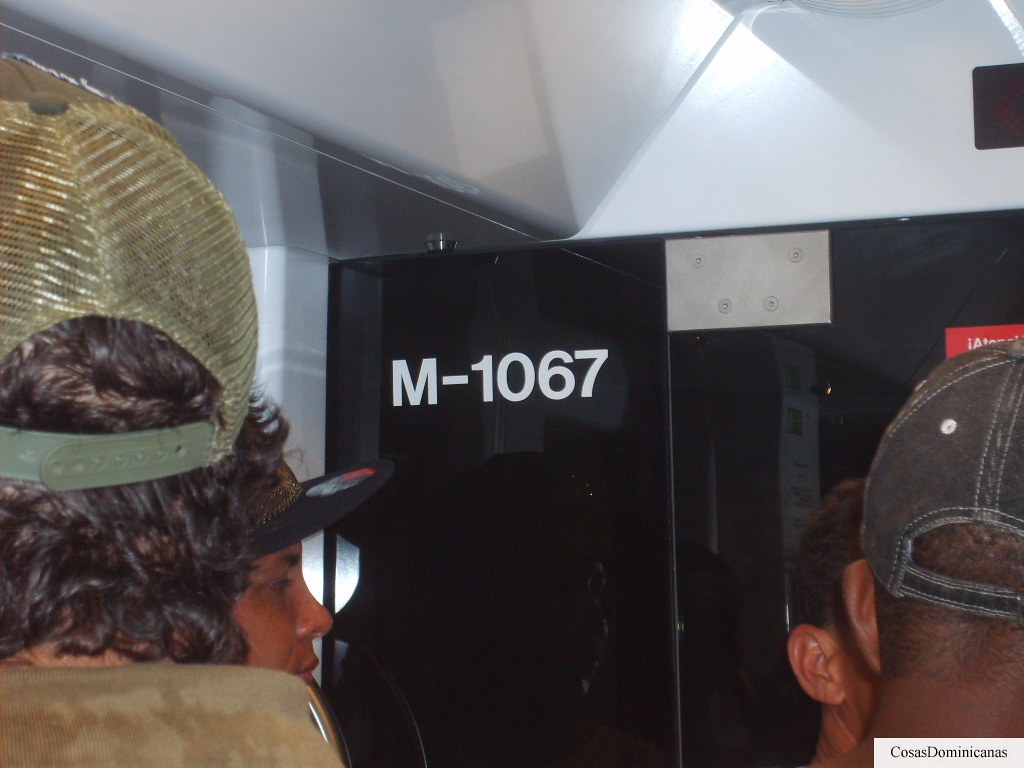In this indoor photograph, likely taken inside a vehicle such as a bus or train, we observe a detailed setting and several individuals. The image is slightly wider than it is tall. Dominating the top portion is a light gray metal ceiling with a distinctive overhang in the upper left, featuring a small key slot. Below, the ceiling line dips towards the center before rising again, framing the space and leading our eye to the focal points.

To the center-right, a reflective black wall is visible, adorned at the top with a metal plate secured by four hex screws. The plate is marked with the text "M-1067" in white. Adjacent to this, a red sticker with white text, partially obscured, adds a splash of color.

In the lower left corner, the back of a man’s head is visible. He has dark brown skin and wears a greenish-brown baseball cap with short, curly black hair extending to the nape of his neck. Slightly shorter and in front of him, another person with dark skin and partial facial profile is seen, also wearing a black baseball cap. Their image is faintly reflected on the black wall ahead.

The lower right corner of the image contains another crucial detail: the text "Cosas Dominicanus," enclosed within a gray box. This accompanies another man positioned with his back to the camera. He has short black hair shaved up the sides and wears a black ball cap with white stitching. In front of him stands a shorter individual, similarly dark-skinned and capped, with their hair just visible from behind the ear.

The color palette of the photograph includes white, black, gray, brown, red, tan, and silver, contributing to the detailed and vibrant indoor scene amidst the varied architectural and human elements.